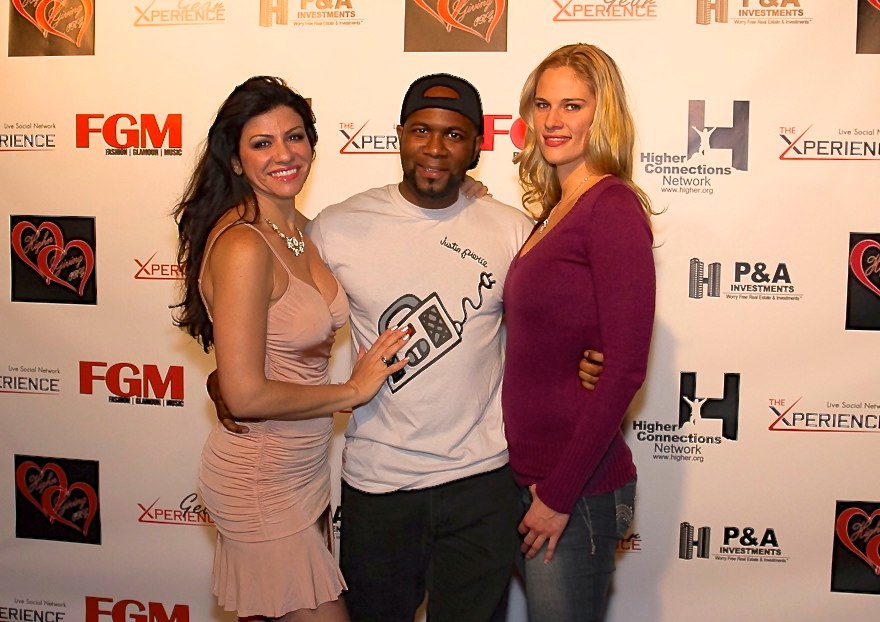The photograph depicts three individuals standing in front of a promotional backdrop featuring logos from FGM, The Experience, Higher Connections Network, and P&A Investments. From left to right, the first individual is a woman with long dark hair, wearing a fitted peach or light-pink dress and a chunky silver necklace. She is smiling widely and has a hand placed on the stomach of the man next to her. The man in the middle, who is Black, is dressed in a white shirt adorned with an illustration of a boombox, a backwards black baseball cap, and black jeans. He has his arms around both women. The woman on the right is notably taller, has long blonde hair cascading past her shoulders, and wears a form-fitting dark purple sweater with jeans. She also sports a necklace and, like the others, is smiling warmly at the camera. The setting hints at an event or possibly a charity function given the branded backdrop and the casual but coordinated attire of the individuals.